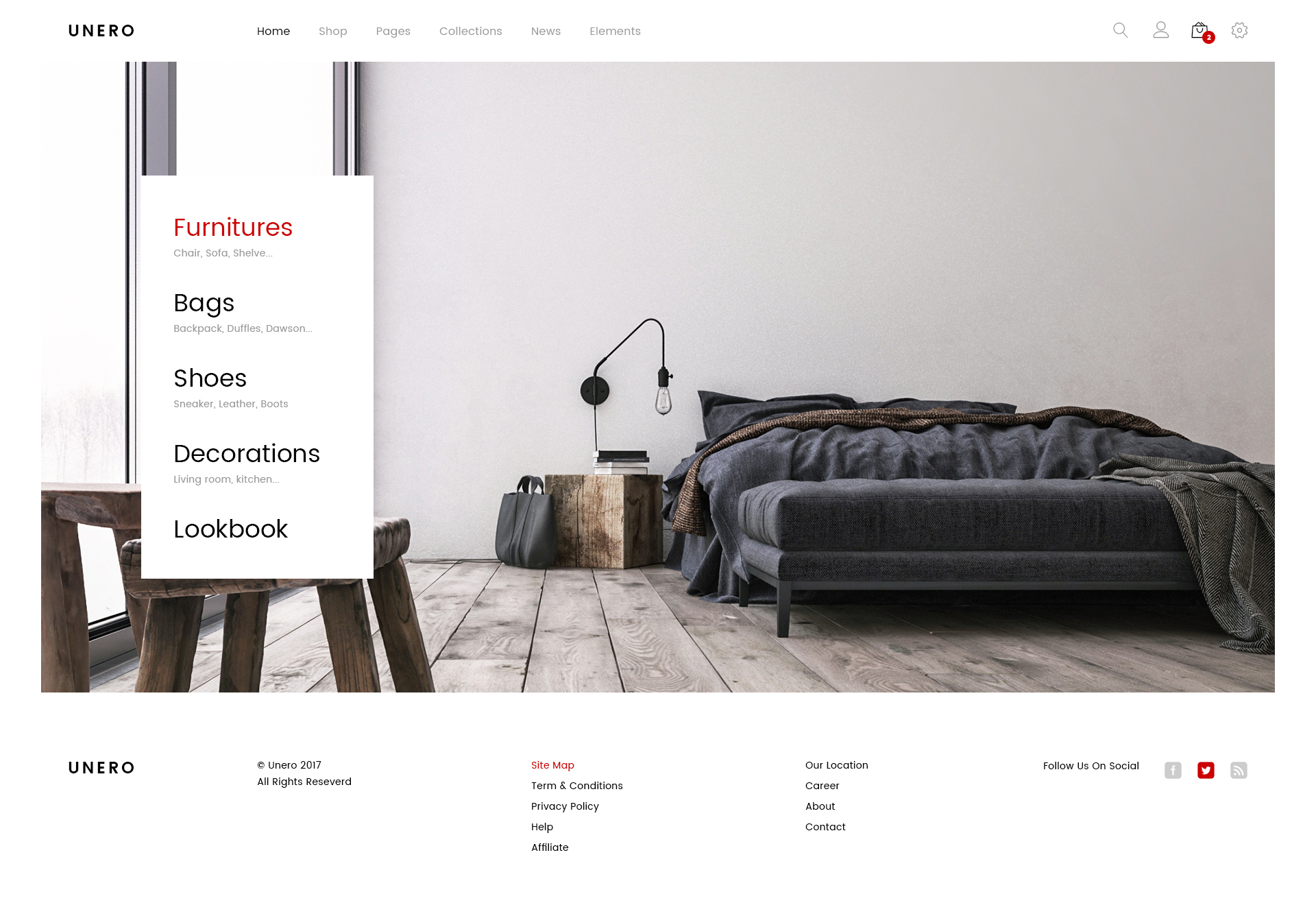Screenshot from the UNERO Website Homepage

This detailed screenshot showcases the homepage of the website "UNERO." At the top of the page, a horizontal menu bar is visible with the following options: Home (selected), Shop, Pages, Collections, News, and Elements. To the top right of the screen, there are icons for Search, Account, Shopping Bag, and Settings.

The background photograph features a minimalist bedroom setup. Positioned near the right side of the image is a large bed adorned with a dark blue blanket that has been casually pulled back. At the foot of the bed is an upholstered bench, adding to the room’s understated elegance. On the left side of the bed, a wooden nightstand is visible, topped with a stack of books and illuminated by a pendant-style lamp. A black tote bag leans against the nightstand, contributing to the room's cohesive design. The bedroom floor consists of wooden planks and the walls are bare, enhancing the minimalist aesthetic.

To the left side of the screenshot, there is a vertical menu with "Furniture" selected. Other menu options include Chair, Sofa, Shelves, Bags, Backpack, Duffels, Dawson, Shoes, Sneaker, Leather, Boots, Decorations, Living Room, Kitchen, and Lookbook.

At the bottom of the page, the footer contains various links: UNERO 2017 All Rights Reserved, Sitemap, Terms and Conditions, Privacy Policy, Help, Affiliate, Our Location, Career, About, Contact, followed by icons for Facebook and Twitter, inviting users to follow UNERO on social media.